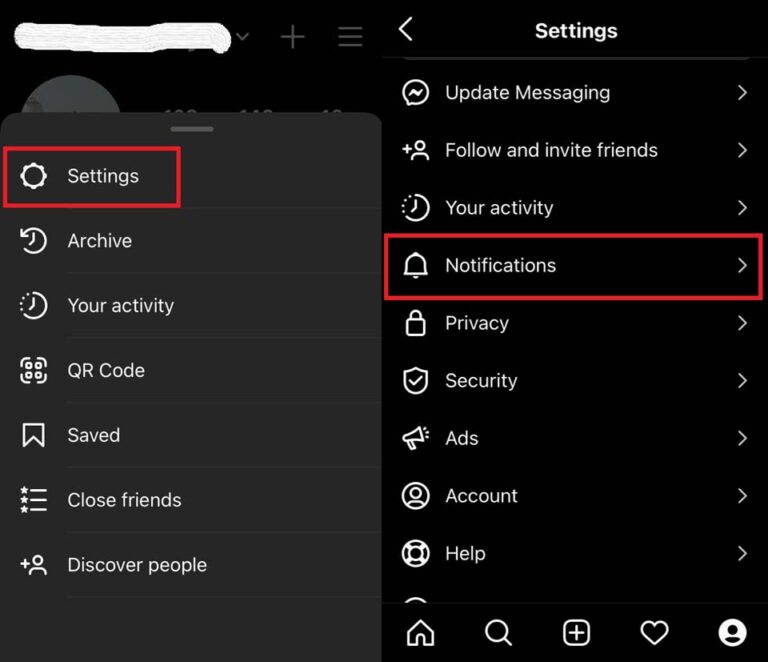The image comprises two side-by-side screenshots of a mobile application interface. The left screenshot depicts a user navigation menu with options such as Settings (highlighted with a red box), Archive, Your Activity, QR Code, Save, Close Friends, and Discover People. The username has been redacted using a paint program. Upon clicking the Settings option, the user is taken to the screen depicted on the right. This second screenshot features the Settings menu with a back arrow at the top, indicating a return to the previous menu. The Settings options listed include Update Messaging, Follow and Invite Friends, Your Activity, Notifications (highlighted with a red box), Privacy, Security, Ads, Account, and Help. Additionally, at the bottom of this screen, there are quick access icons for Home, Search, Add (plus sign), Activity (heart), and Profile (person icon, possibly for contacts).